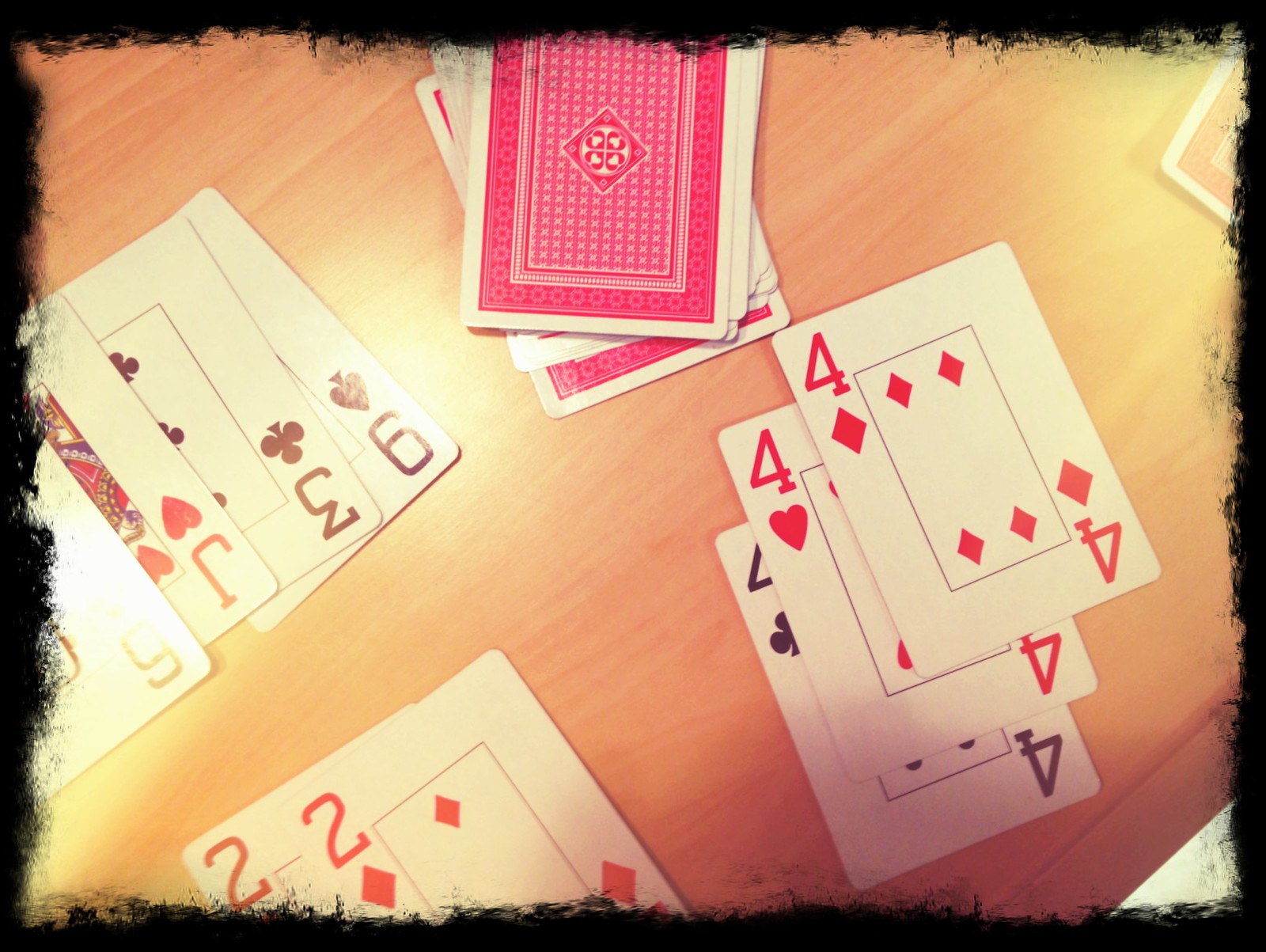This photograph captures a spontaneous arrangement of playing cards on a blonde wooden table. The image features a unique, black smoky, and distorted border that gives it an artistic and surreal frame. Light reflections play across the smooth surface of the table and onto the cards, adding a touch of vividness to the composition.

The playing cards are predominantly white, adorned with intricate pink floral motifs and pink checkered borders, exuding an elegant, old-world charm. They are scattered about—with some face-up and others face-down, creating an element of casual disorder. Noteworthy among the face-up cards are a red Four of Diamonds, a red Four of Hearts, a black Four of Clubs, a red Two of Diamonds, another red Two, a Nine of Spades, a Three of Clubs, and a red Jack of Hearts. One card's face is partially obscured by a bright camera flash, making it impossible to distinguish the suit of the six visible.

A small, subtle spot of a white surface peeks from the bottom corner of the photo, adding an extra layer of intrigue to the scene. The overall aesthetic of the photograph is described by washed-out colors and an over-focused, oversaturated look, lending it an almost dreamlike, vintage quality.